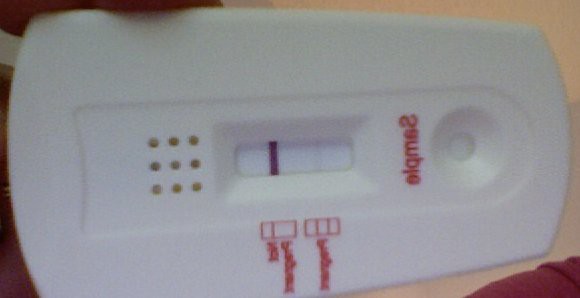The photograph depicts a white, rectangular diagnostic test device, oriented in a manner that suggests the image might be a reflection. The test device features an indented area at its center, containing an array of nine dots arranged in a 3x3 square pattern. Adjacent to these dots on the right side is a small rectangular window displaying a single purple line.

To the left of the window, the text appears reversed, readable as "SEMBLE." Additionally, nearby is a designated circular area likely intended for the application of liquid samples.

At the bottom of the image, beneath the testing window, there are two additional rectangular sections. The left rectangle contains one line and some unreadable text below it, whereas the right rectangle displays two lines. This likely indicates that one line represents a negative result and two lines signify a positive result.